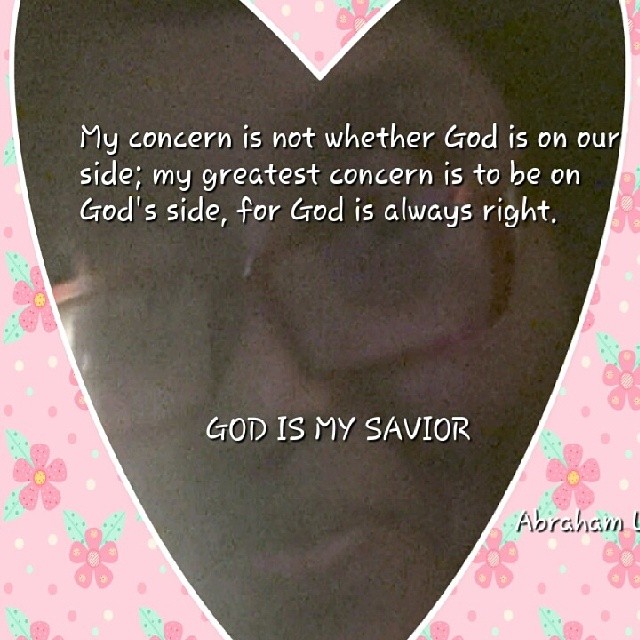This image is a square-shaped, Christian inspirational poster set against a light pink background adorned with five-petaled pink flowers featuring yellow or pink centers and light mint green leaves. The centerpiece is a large, black heart with narrow tips that extend off the top of the image, while the bottom point is out of view. The heart has a thin white outline. In the upper section of the heart, white text reads: "My concern is not whether God is on our side; my greatest concern is to be on God's side, for God is always right." Below this, centered within the heart, it says in all caps, "GOD IS MY SAVIOR." In the lower right-hand corner, "Abraham" is written in white.

Upon closer inspection, the black heart isn't plain; it subtly reveals the reflection of a woman, possibly of African descent, wearing square glasses. This nuanced detail becomes apparent only after focusing on the heart's surface. The overall design merges spiritual messaging with a floral aesthetic, creating an evocative and reflective piece.